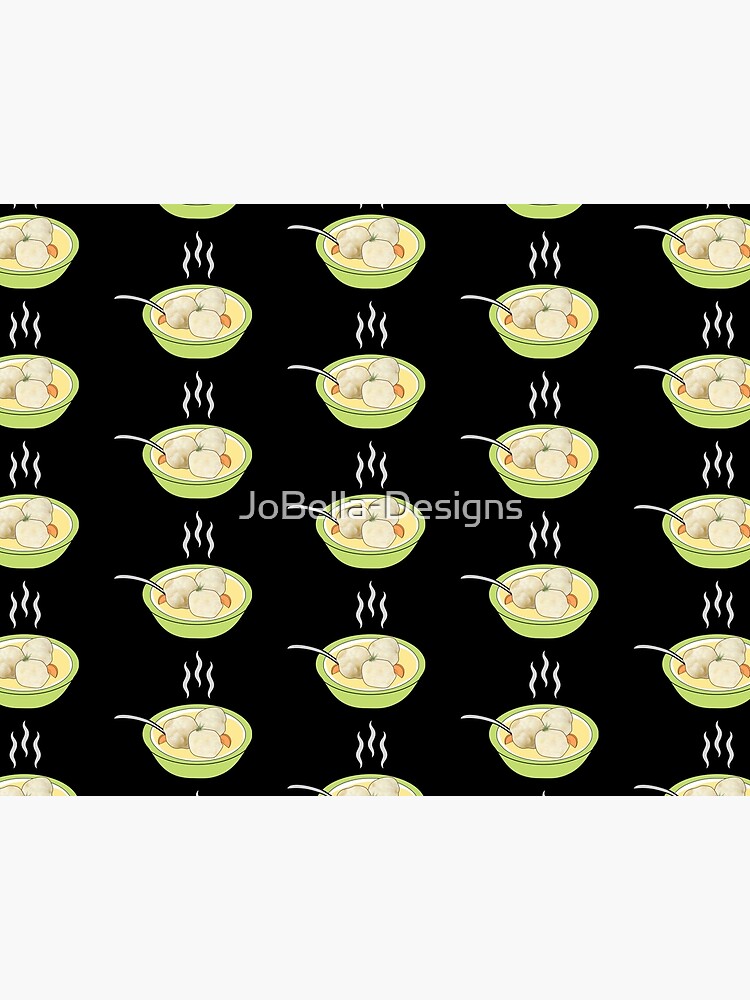The image is a detailed digital drawing with a black background, featuring a repeating pattern of green bowls filled with a creamy, yellowish soup, possibly containing dumplings. Each bowl has a spoon sticking out from the left side and is accompanied by two small orange pieces, which might be carrots or slices of another orange-colored ingredient. Rising from each bowl are three wiggly lines of steam, indicating the soup's warmth. The pattern is arranged in rows, with about four to five bowls in each row, and the layout alternates between rows of three and rows of two bowls. In the center of the design, there is a watermark that reads "Joe Bella Designs". This detailed and neatly arranged pattern gives it the look of a fabric design or wrapping paper, suitable for various background applications.